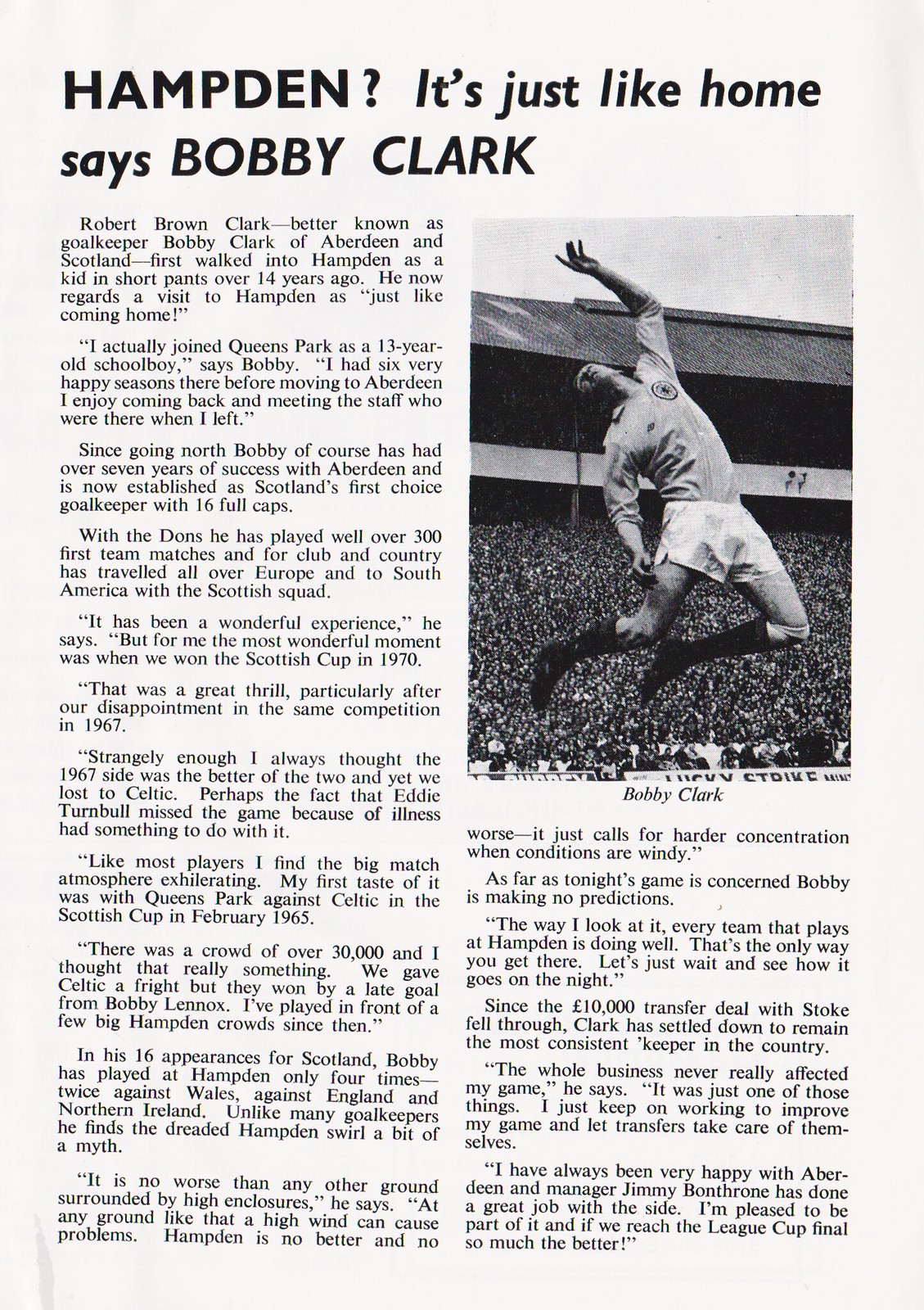This image depicts a black-and-white photo scanned from a publication, likely a book or a magazine, featuring a detailed article about Bobby Clark, the renowned Aberdeen and Scotland goalkeeper. At the top of the page, the headline reads, "Hampton? It's just like home, says Bobby Clark." The page is divided into two primary columns of text. The left column spans the entire length of the page, while the right column is narrower and positioned below a photograph.

The photograph shows Bobby Clark in action, capturing the goalkeeper leaping into the air with his left arm extended upwards and the other arm down, set against a backdrop of a packed stadium. Below this image, his name, "Bobby Clark," is written in italicized black text.

The article begins with an introduction to Robert Brown Clark, more commonly known as Bobby Clark, reminiscing about his first visit to Hampton over 14 years ago as a schoolboy. He describes Hampton as feeling just like home. It details his journey from joining Queen's Park at thirteen, experiencing joyful seasons there, and eventually moving to Aberdeen.

The text highlights his successful career—spanning over seven years with Aberdeen, competing in more than 300 matches for both club and country, and earning 16 caps for Scotland. Significant moments such as winning the Scottish Cup in 1970 and narrowly missing victory in 1967 are noted, along with his lively account of playing in front of large crowds at Hampton.

Bobby also comments on the so-called "Hampton swirl," dismissing it as a myth, citing that any stadium with high enclosures can cause wind issues, which requires increased concentration. Reflecting on his career, he expresses contentment with Aberdeen and the leadership of manager Jimmy Bonthrone, while maintaining his focus on improving his game, unaffected by transfer speculations.

The narrative concludes with Bobby's anticipation of a forthcoming match at Hampton, emphasizing the unpredictability of the game's outcome. Throughout the piece, Bobby's deep connection to Hampton and his gratitude for his remarkable career are evident.